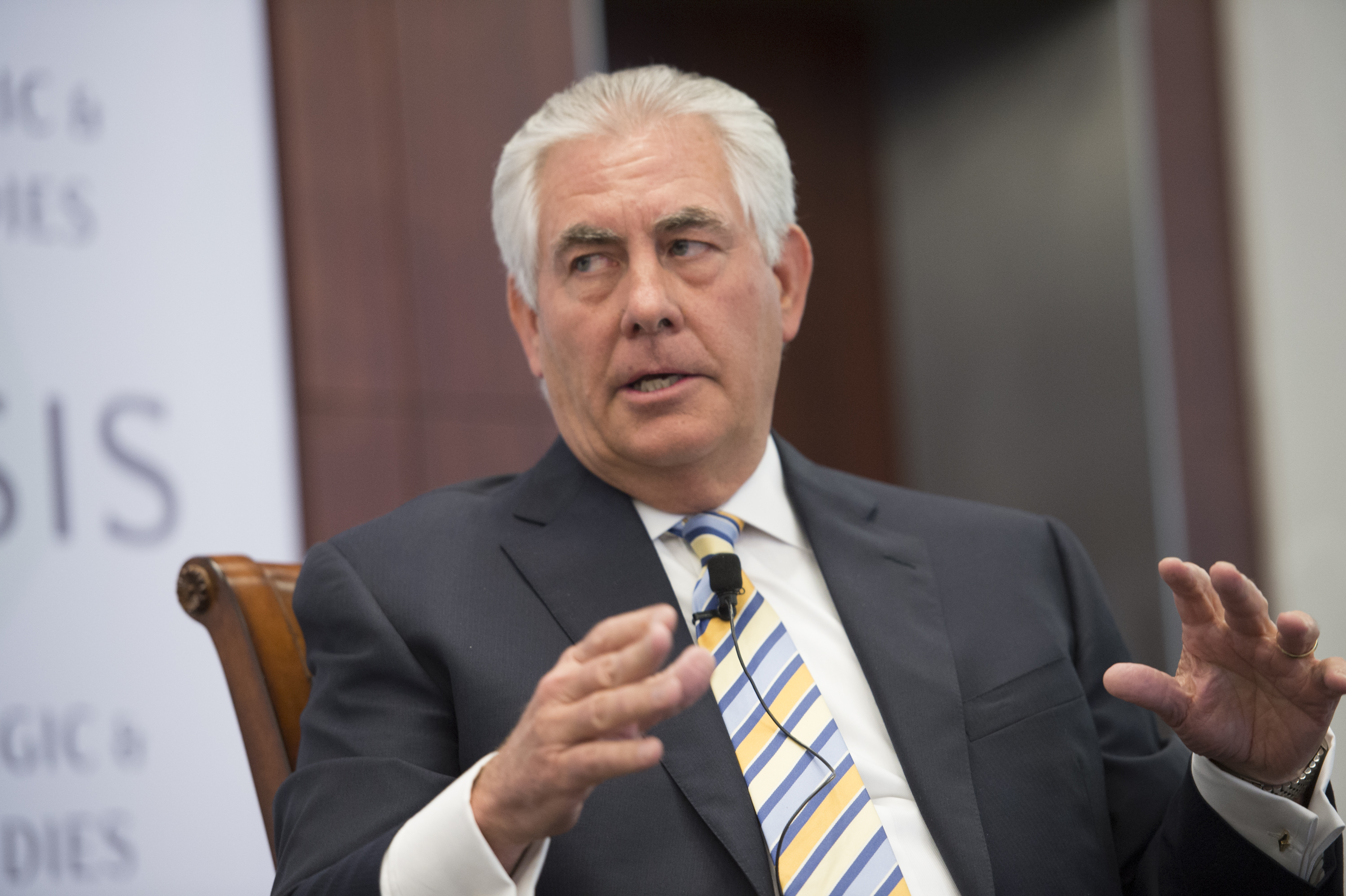The image features an older man, around 70 years old, seated in a chair with a brown wooden backrest. He has short white hair and is dressed in a dark gray suit jacket. A microphone is attached to his tie, which features a repeating diagonal stripe pattern of yellow, blue, white, light blue, and navy blue. Underneath his jacket, he wears a white button-up shirt with white cuffs and cuff links visible. The man holds his hands in front of him, gesturing as if explaining something, and you can also see the links of a watch on his left wrist. He is looking to the right, engaged in conversation. Behind him is a blurry scene with an open door to the right and a partially visible white poster or banner with unreadable text on the left.